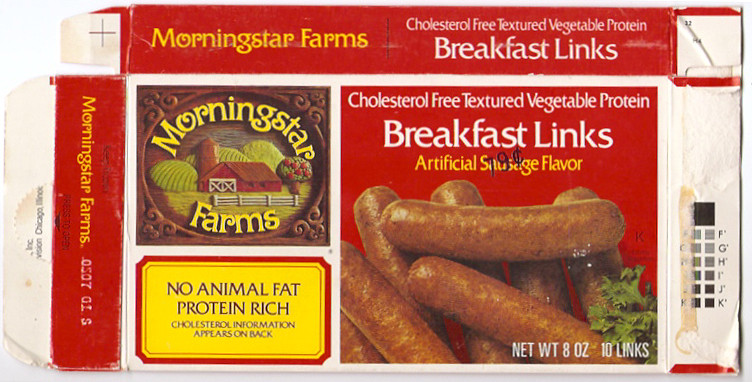Caption: 
An 8-ounce pack of Morning Star Farms breakfast sausage links, containing a total of 10 links. These sausage links are made from vegetable protein, making them a meat-free alternative with no animal fat. Rich in protein, they are labeled as "low in electricity sausages" and are priced at just $0.79.